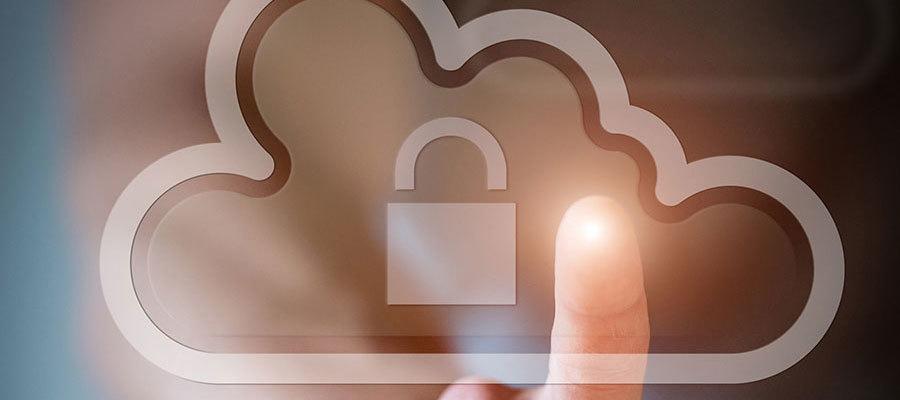The image prominently features a clear, close-up logo of a translucent cloud commonly used to represent cloud storage. The cloud is outlined in black and white and has a padlock icon inside it, emphasizing security. There is a white person’s finger, illuminated at the tip, seemingly interacting with the cloud logo as if it's a touchscreen icon. The background is predominantly brown with a blur that lacks detailed shapes, creating a stark contrast with the brightly lit finger and the cloud logo in the center. The setting is well-lit, making the cloud logo and the finger's interaction the focal points of the image. No words or additional objects are present in the scene.